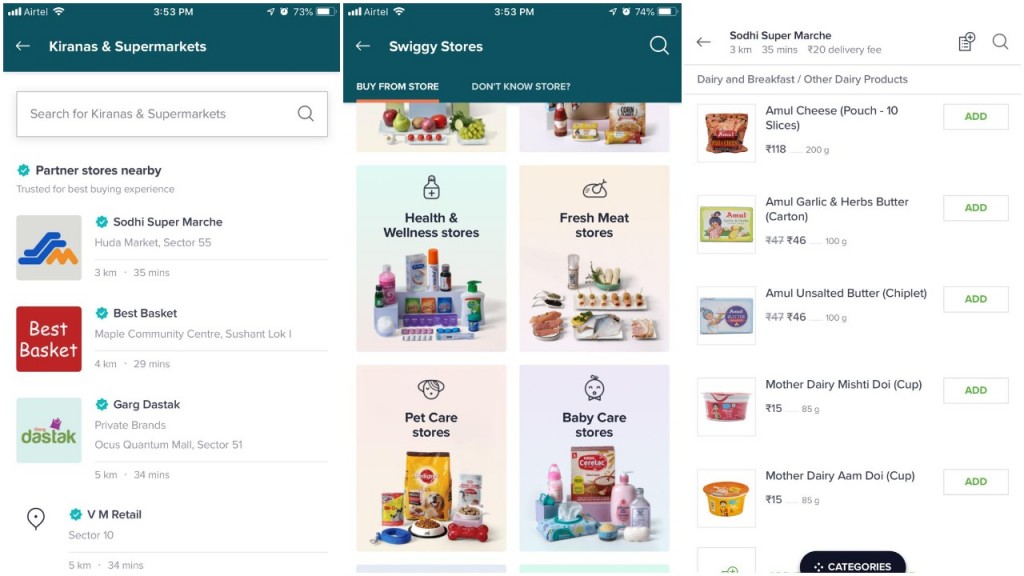The image appears to be a screenshot from a mobile app designed to help users locate and browse various types of stores, similar to a supermarket directory. On the left side of the screen, there are three distinct sections with the titles: "Kiranas," "Supermarkets," and a search bar labeled "Partner Stores Nearby." Beneath this, three specific stores are listed: "Sodhi Marche," "Best Basket," and "Garg Dust Stock," indicating a foreign setting.

In the middle of the screen, a highlighted section titled "Swiggy Stores" is visible, showcasing categorized store options such as health and wellness stores, fresh meat stores, pet care stores, and baby care stores, each represented by corresponding images.

On the right side of the screen, the user has specifically selected "Sodhi Marche," revealing a variety of items under their "Other Dairy Products" section. The detailed layout and categorization suggest that the app provides a comprehensive and user-friendly way to explore and shop at different types of stores.